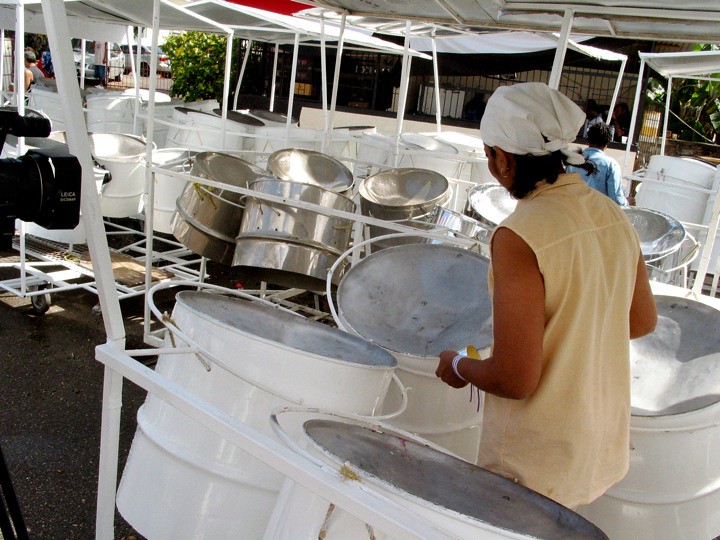This rectangular outdoor photograph captures a lively scene dominated by an arrangement of steel drums under a covered area. The space is bordered with black wrought-iron fencing from floor to ceiling. Most of these drums are organized into groups of four, each set framed by a white metal structure with an individual roof. The majority of the drums feature a white exterior and silver tops, except for two sets in the center, which are entirely stainless steel in color.

On the right-hand side of the image, a person stands inside one of these drum sets, seemingly prepared to play. This individual has long, dark hair partially covered by a white scarf or bandana and wears a yellow sleeveless shirt. The precise identity and gender of this person are ambiguous due to the obscured face.

To the far right, the photo shows a small building and some tents housing additional drum sets, indicative of a market or display area typical in the Caribbean. The upper left corner reveals a figure in the background clad in a gray sleeveless shirt. The scene suggests a vibrant, musical atmosphere, with white tables and chairs in the background for alfresco dining, enhancing the lively, communal ambiance.